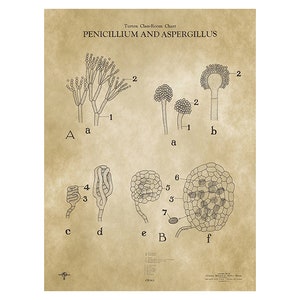The illustration titled "Penicillin and Aspergillus" features detailed, aged biological diagrams on a browned, eight and a half by eleven piece of paper. The diagrams are annotated with various letters and numbers. At the top left, the image labeled 'A' depicts two stalk-like structures comprised of several shorter segments topped with multiple ball-shaped objects, representing Penicillium. Adjacent to it on the upper right, the diagram labeled 'B' showcases a thicker stalk, capped with numerous small, round components. The bottom right corner has two structures, resembling a human colon, labeled 'C' and 'D'. Overall, the detailed pen-and-ink line drawings demonstrate the branching Y-shaped structure of Penicillium and the segmented, winding form of Aspergillus. Both fungi are identified by specific labeled sections ranging from A to F and are associated with numbers for additional detail.